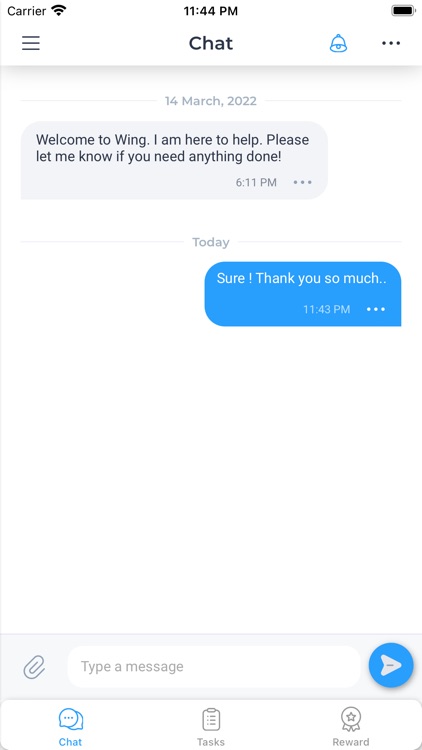The screenshot displays a chat app interface on a smartphone with a white background. The top toolbar shows the carrier signal strength with three bars on the left, the time "11:44 PM" in the center, and a nearly full battery icon (99-100%) on the right. Below this toolbar, the app's header reads "Chat" in the center, flanked by a blue bell icon on the right and three horizontal dots, indicative of a menu, on the far right. On the left side of the "Chat" header, there are three vertical gray bars, suggesting additional menu options.

Within the body of the chat, a date stamp reads "14th March 2022." The first message, sent at "6:11 PM," states: "Welcome to WEAN. I am here to help. Please let me know if you need anything done." A reply, timestamped "Today" at "11:43 PM," is in a blue bubble and reads: "Sure, thank you so much."

At the bottom of the screen, there is a text input field for composing messages, accompanied by a blue circle on the right containing a white paper airplane icon, which acts as the send button.